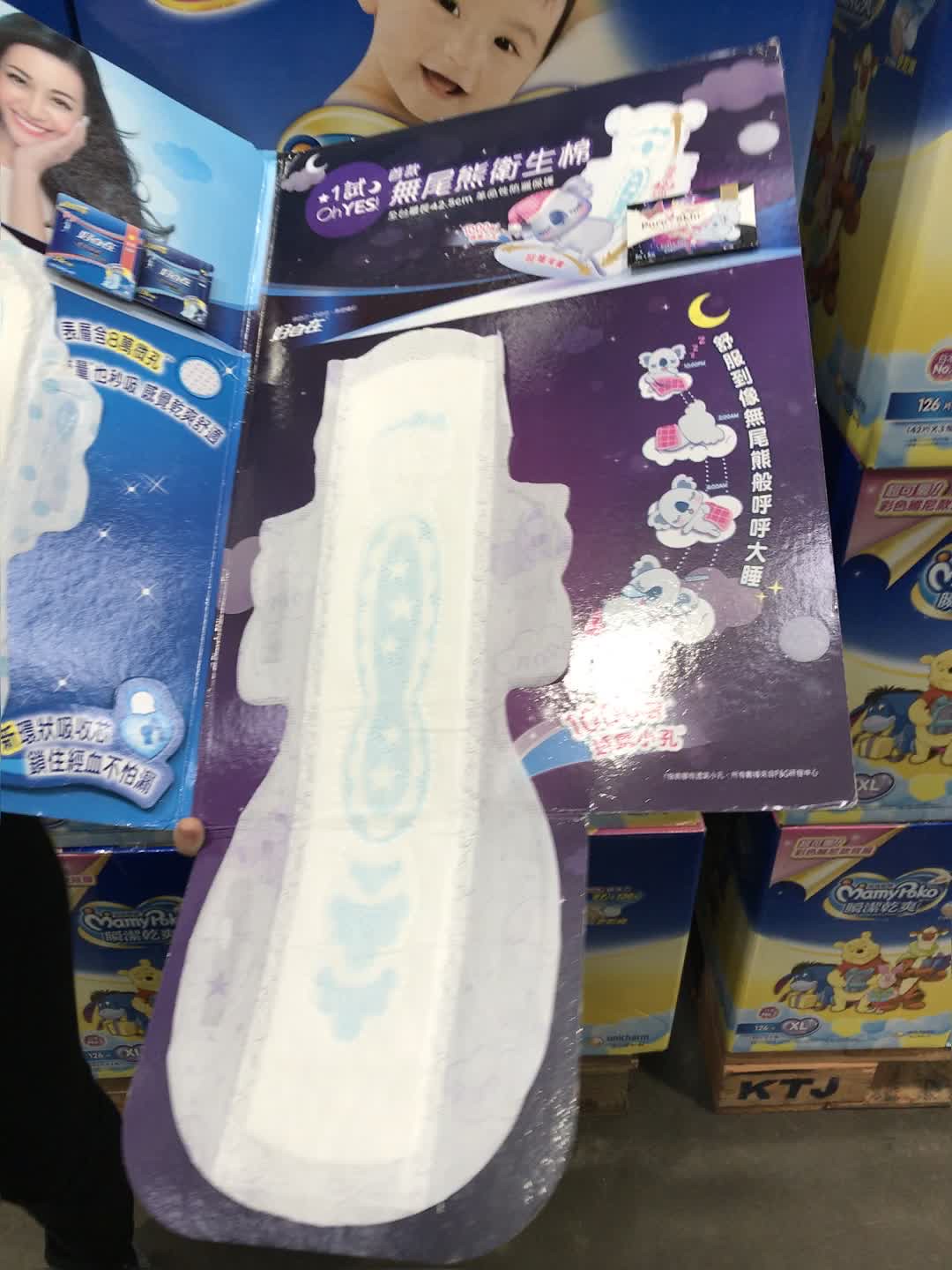The image depicts a section of a store aisle, possibly in a toy or hygiene products section, with a concrete or brown carpeted floor. Central to the image is an open booklet featuring a promotional sanitary or hygiene pad. The pad, set against a purple background with stars suggesting the night sky, has a white outline shaped somewhat like a bear and showcases a sleeping koala logo in a pink nightcap, emphasizing its softness and comfort.

Surrounding the booklet are several stacked boxes of similar products. On the right side, there's a light blue box with an image of a woman with long hair resting her face in her hands. Above it, another box features the face of a baby looking sideways. At the bottom of the stack, a crate marked "KTJ" holds more boxes, one of which is decorated with characters from Winnie the Pooh—Tigger, Piglet, and Eeyore.

Additionally, a person's leg stepping away is visible in the background, indicating the presence of shoppers. This setting likely mixes colorful, child-friendly branding with adult hygiene product promotional displays, creating a vivid and detailed scene.